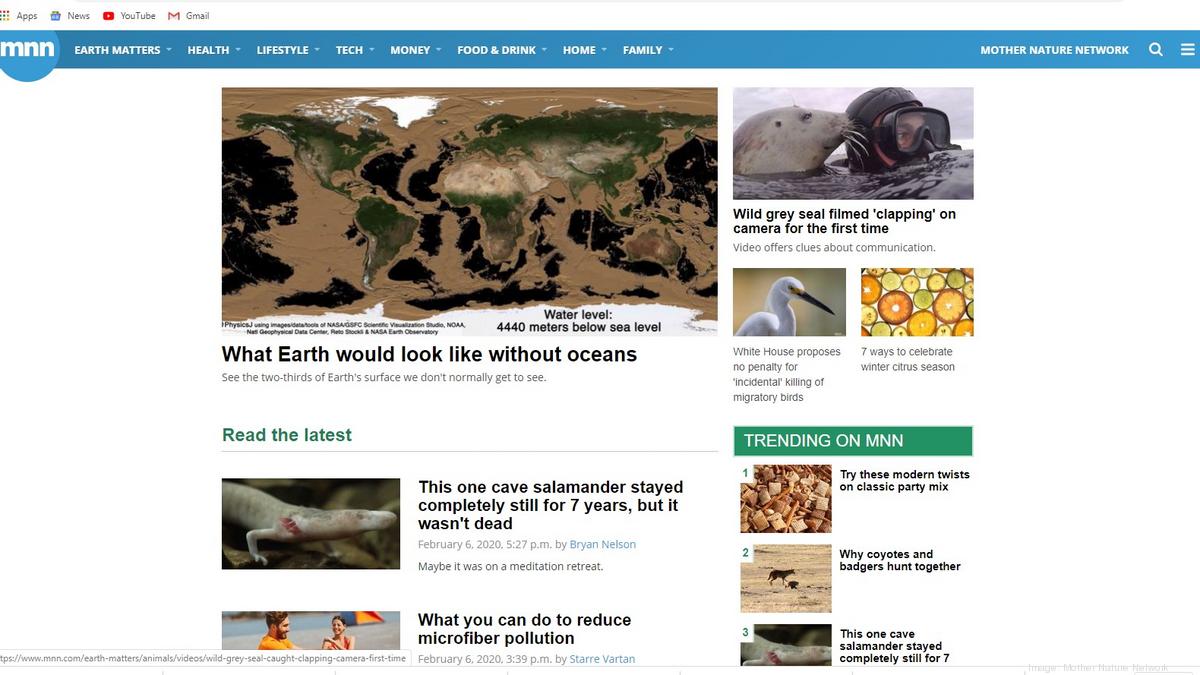The image depicts a small and blurry web page that necessitates zooming in to read the details. At the top of the page, the navigation menu features tabs labeled "Apps," "News," "YouTube," and "Gmail," as well as a bookmark bar. There is a blue border with an "MNN" logo inside a circle. 

Beneath this, drop-down menus include categories such as "Earth Matters," "Health," "Lifestyle," "Tech," "Money," "Food and Drink," "Home and Family," and "Mother Nature Network." 

On the main section of the page, various articles are displayed. One prominently features an image of the Earth, showing brown land where oceans are usually depicted. The article headline reads, "What Earth Would Look Like Without Oceans," with a subheading stating, "Water level 4,440 meters below sea level," and further text inviting readers to "see the two-thirds of Earth's surface we don't normally get to see."

To the right, another article is titled, "Gray Seal Filmed Clapping on Camera for the First Time," noting that the video offers new insights into communication. Another nearby headline reads, "White House Proposes No Penalty for Incidental Killing of Migratory Birds."